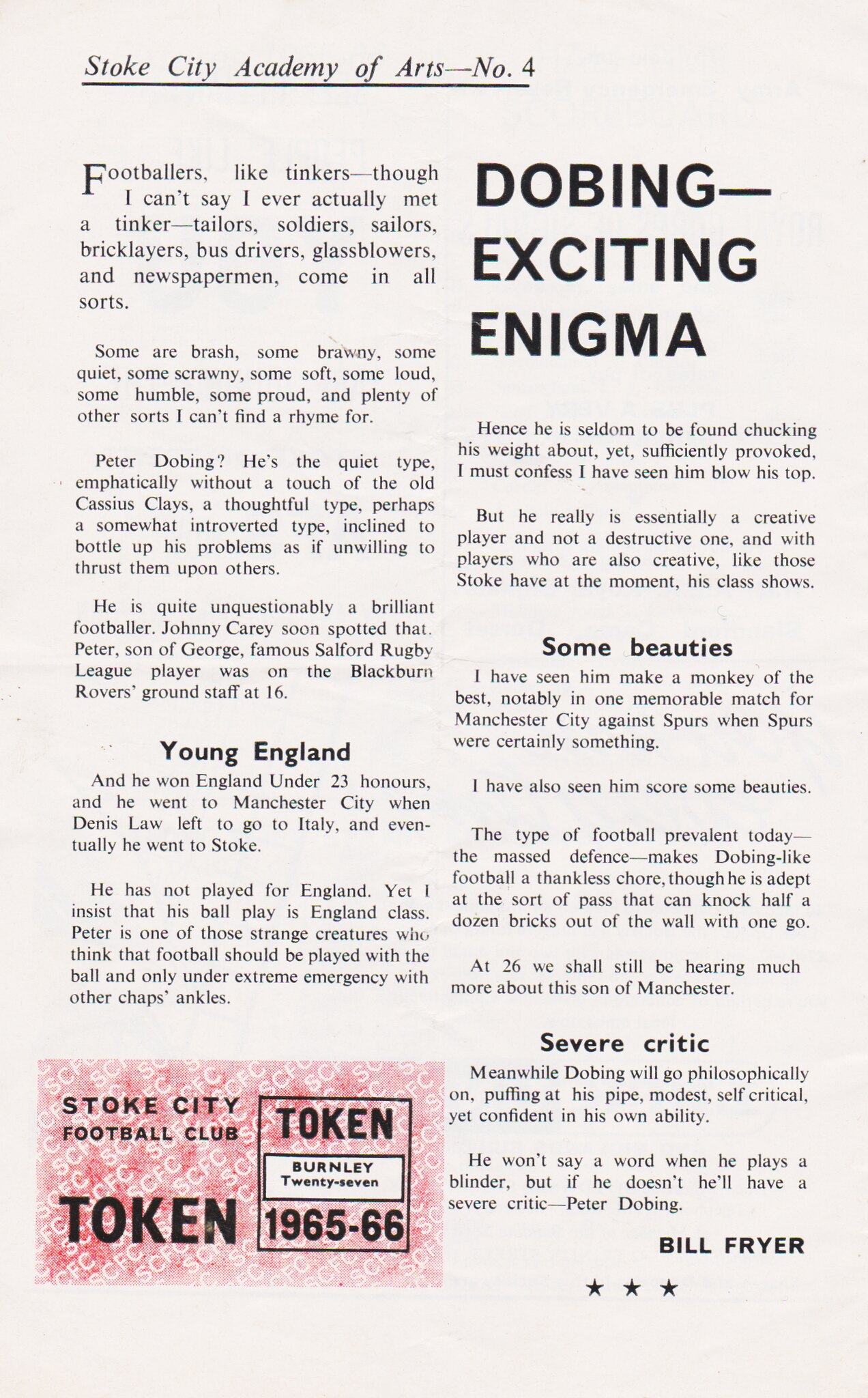The image is a scanned page from a magazine, predominantly showcasing articles on the Stoke City Football Club, specifically focusing on their Academy of Arts, issue number four. The page features multiple columns of text, starting with an underlined header "Stoke City Academy of Arts number four." A significant portion of the page discusses various personalities in football, including a detailed description of Peter Dobing, highlighting his thoughtful and introverted nature. Key phrases such as "footballers like tinkers, though I can't say I've ever actually met a tinker" introduce a poetic list of different types of people involved in sports. The columns are interspersed with headings such as "young England," "some beauties," and "severe critic."

On the top of the right-hand column, the text "DOBING: EXCITING ENIGMA" appears in all capital letters. Bill Fryer is credited as the author, and his name is followed by three black stars in a horizontal row positioned at the page's bottom right. Additionally, there is a small advertisement for the Stoke City Football Club in the bottom left of the page, featuring a red background and details about a token for the 1965-66 season. The detailed, poetic descriptions and the various sections contribute to a rich, multi-faceted portrayal of the football culture and personalities associated with Stoke City.